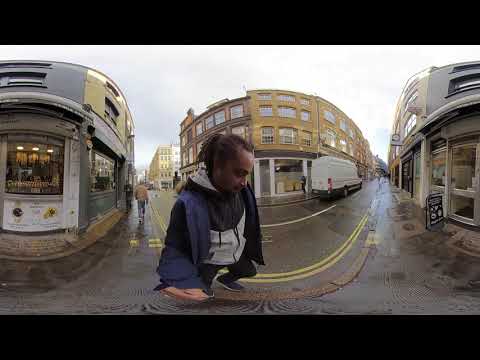In this intricate and surreal image captured with an extreme fisheye lens, a young man with a ponytail is squatting in the center of an intersection in a downtown area. He is dressed in layered clothing, consisting of a blue hoodie over a black jacket, paired with dark pants and sneakers. The scene gives the impression of two photographs seamlessly stitched together, enhancing the panoramic effect and making two intersecting streets appear parallel. The overcast sky casts a muted light over the surroundings, hinting at recent rain visible on the ground.

Surrounding the man, three distinct buildings come into view. On one side, a busy cafeteria or store displays its menu on the street, attracting a few pedestrians. To his right, another similar establishment adds to the urban ambiance. The central building, a modern glass-fronted structure spanning three to four stories, stands prominently behind him. Additionally, wagon-like structures reminiscent of railroad cars flank the scene. The streets stretch beyond the center, populated with a diverse array of people, adding a bustling vibe to the downtown area, which may be located in a foreign country suggested by unrecognizable text on a mirror.